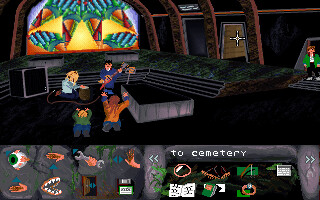This image is a detailed screenshot from a video game, depicting a dramatic scene set in a room that resembles a church's attic. The focal point of the scene is a large, colorful stained-glass window at one end of the room, featuring vibrant hues of yellow, green, blue, red, and orange. Below the window is a black floor, where a large speaker is placed. The speaker is connected by a cord to a red electric guitar, held by a male character in a blue trench coat. This character appears to be playing the guitar. 

Next to him is a kneeling individual wearing a light blue shirt and headphones, whose actions are unclear but who seems engaged in the activity. In front of these two characters, there are two individuals who appear to be either cheering or begging, their arms raised. One of them, a blonde, wears a green shirt, while the other, with long brunette or possibly red hair, sports an orange shirt. 

On the far right of the room, a person in a green jacket and white shoes stands near an opening by a door equipped with a vault-like handle, reminiscent of a bank door. The room is framed by brown support pillars and black walls, giving it a gothic and somewhat industrial atmosphere.

At the bottom of the screen are various icons for in-game actions. On the left side, the icons include an eyeball, multiple hands in different gestures, a wrench, a set of teeth, and an open door. On the right side, words read "To Cemetery," accompanied by more icons including a magnifying glass, a book, and other indistinguishable items.

Overall, the image captures a vibrant and complex scene within the game, rich in visual details and interactive elements.